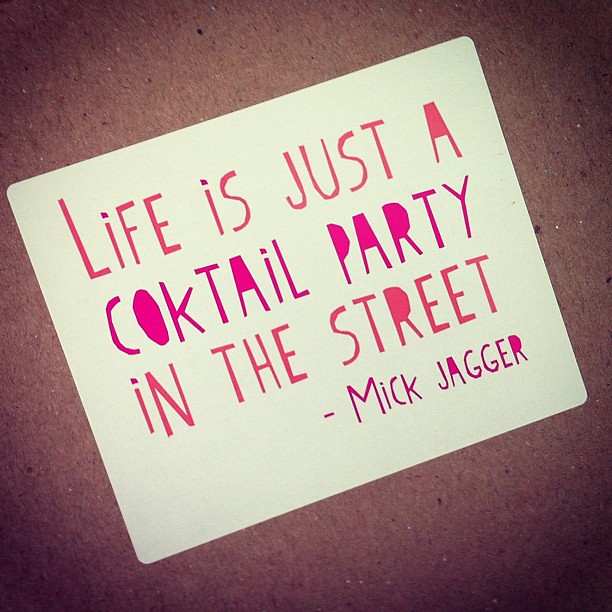The image showcases a single, diagonally oriented white card against a brown, somewhat textured backdrop resembling a cardboard floor, with a sepia filter adding a vintage touch. Positioned centrally, the card bears a quote in an engaging font, where letters with enclosed spaces, like 'A,' 'O,' and 'R,' are fully filled in with color. The text, in alternating shades of light and dark pink, reads: "Life is just a cocktail party in the street." Beneath this, attributed in dark pink, is "Mick Jagger." The vibrant hues of white, pink, and purple contrast with the muted brown background, creating an eye-catching and upbeat visual that feels perfect for social media sharing.